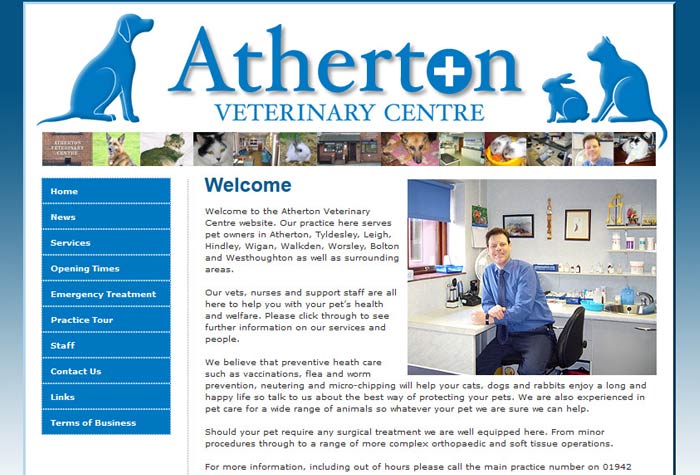This screen capture showcases the landing page of the Atherton Veterinary Centre's website. At the top of the page, the header features the name "A-T-H-E-R-T-O-N" centrally positioned, flanked by a blue silhouette of a dog on the left and silhouettes of a cat and a rabbit on the right. Beneath the name, the text "Veterinary Centre" is displayed, using the British English spelling "C-E-N-T-R-E."

Below the header, a collage spans across the page with images depicting various pets, including cats, rabbits, and dogs. The main section of the page features a welcome message from the veterinarian, accompanied by a photo of the vet. In the image, the veterinarian is seated at a desk, leaning slightly to the right, and looking directly at the camera. He is dressed in a blue shirt and dark black pants, while the background showcases several awards on the wall behind him.

On the left side of the page is a vertical navigation menu with tabs labeled: Home, News, Services, Opening Times, Emergency Treatment, Practice Tour, Staff, Contact Us, Links, and Terms of Business. The web page is visually appealing, with clear, sharp images and a well-organized layout, making it an effective landing page for the Atherton Veterinary Centre.